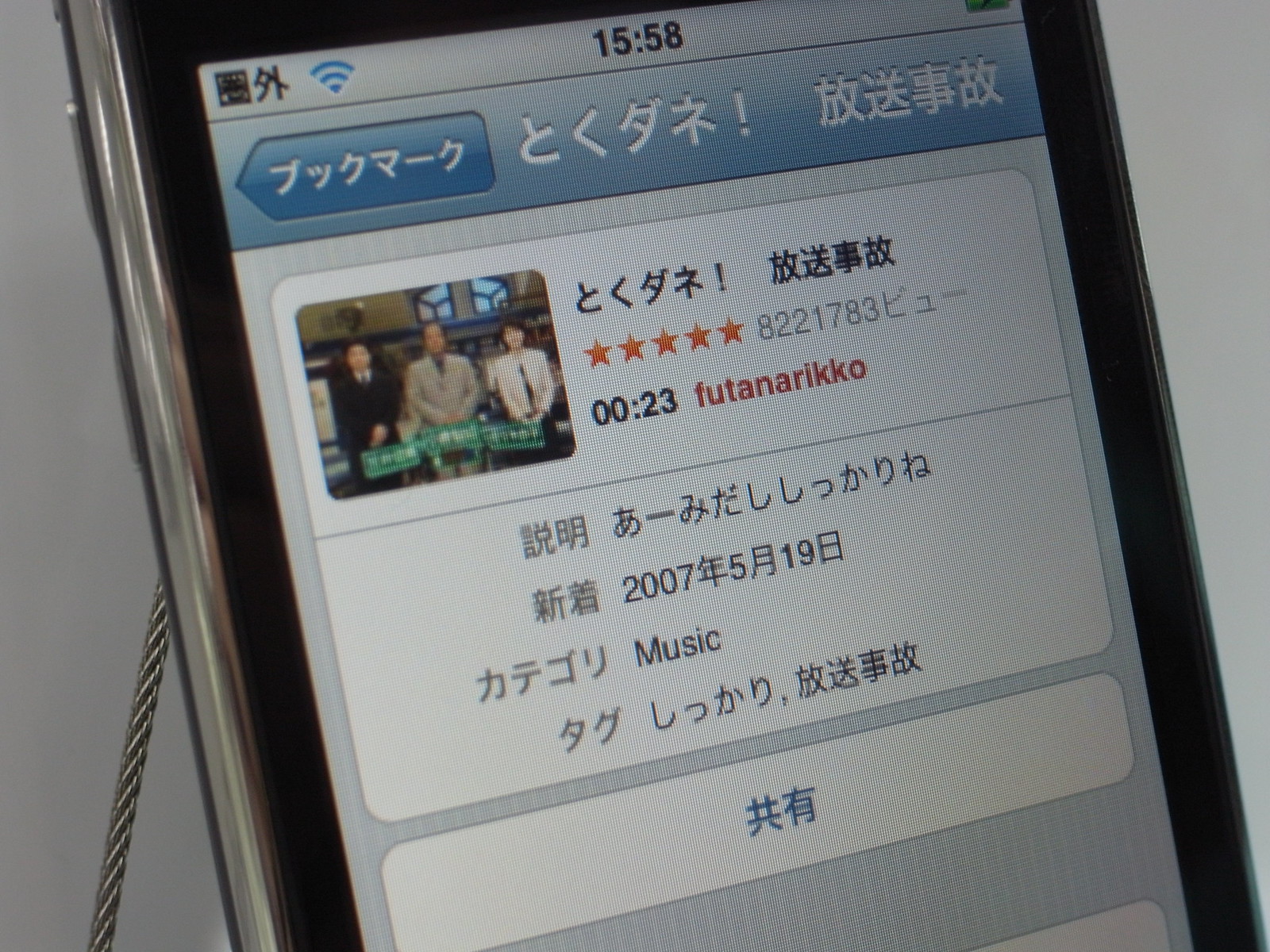This image features a close-up view of a cell phone screen, tilted counterclockwise and zoomed in, revealing only a portion of the display. At the top of the screen, various icons are visible, including the Wi-Fi signal and half circles indicating notifications or volume. The time displayed on the screen is 15:58, written in a digital font.

Beneath the header, there are Asian characters, likely Japanese or Korean, followed by an image of three indistinct people standing at green podiums. The first individual on the left appears to be a male wearing a black suit, the middle figure is a male in a gray suit, and the person on the right is too blurry to identify. Next to the image, there are five orange stars and the text '8221783.' Below, in bold black text, it reads "00:23" with 'FUTANARIKKO' in red lettering adjacent to it.

Continuing down the screen, more Asian characters are displayed, interspersed with identifiable terms such as "music" and '2007 519.' The background at the very bottom shifts to another white box containing additional Asian symbols. A metal braided wire emerges from the device, visible in the lower left section.